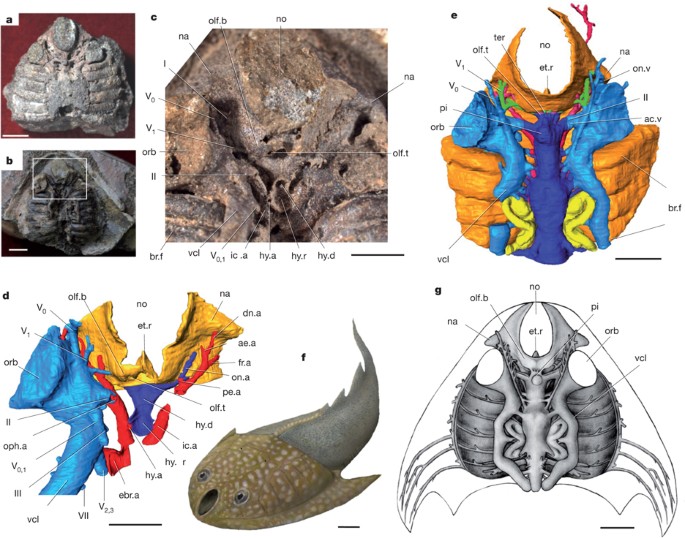The scientific image depicts a detailed study of an ancient fish-like creature, arranged in a series of labeled panels marked A through G. Panels A and B in the top left, feature photographs of the fossilized remains of the organism. Panel C, positioned at the top center, offers a zoomed-in view of a specific fossil section, annotated with bullet points indicating various anatomical features. In the top right, Panel D, there is a 3D diagram illustrating this creature, color-coded in shades of orange, yellow, blue, dark blue, and red, with labels comprising short combinations of letters and numbers like "pi," "V1," and "orb."

At the bottom, Panel E provides another 3D representation, highlighting specific internal organs with similar labels, while Panel F showcases an artist's rendition of the fish. This illustration details the creature's appearance, characterized by large eyes, a big oval-shaped mouth, a semi-snake-like body, serrated fins, and short, stubby fins resembling those of a manta ray, with a body coloration of gray and brown spots. Panel G, located at the bottom right, presents a black-and-white diagram of the fish's anatomical structures, again annotated with multiple labels for scientific reference. These coordinated images collectively offer a comprehensive visualization, mapping the organism's external and internal anatomical features.